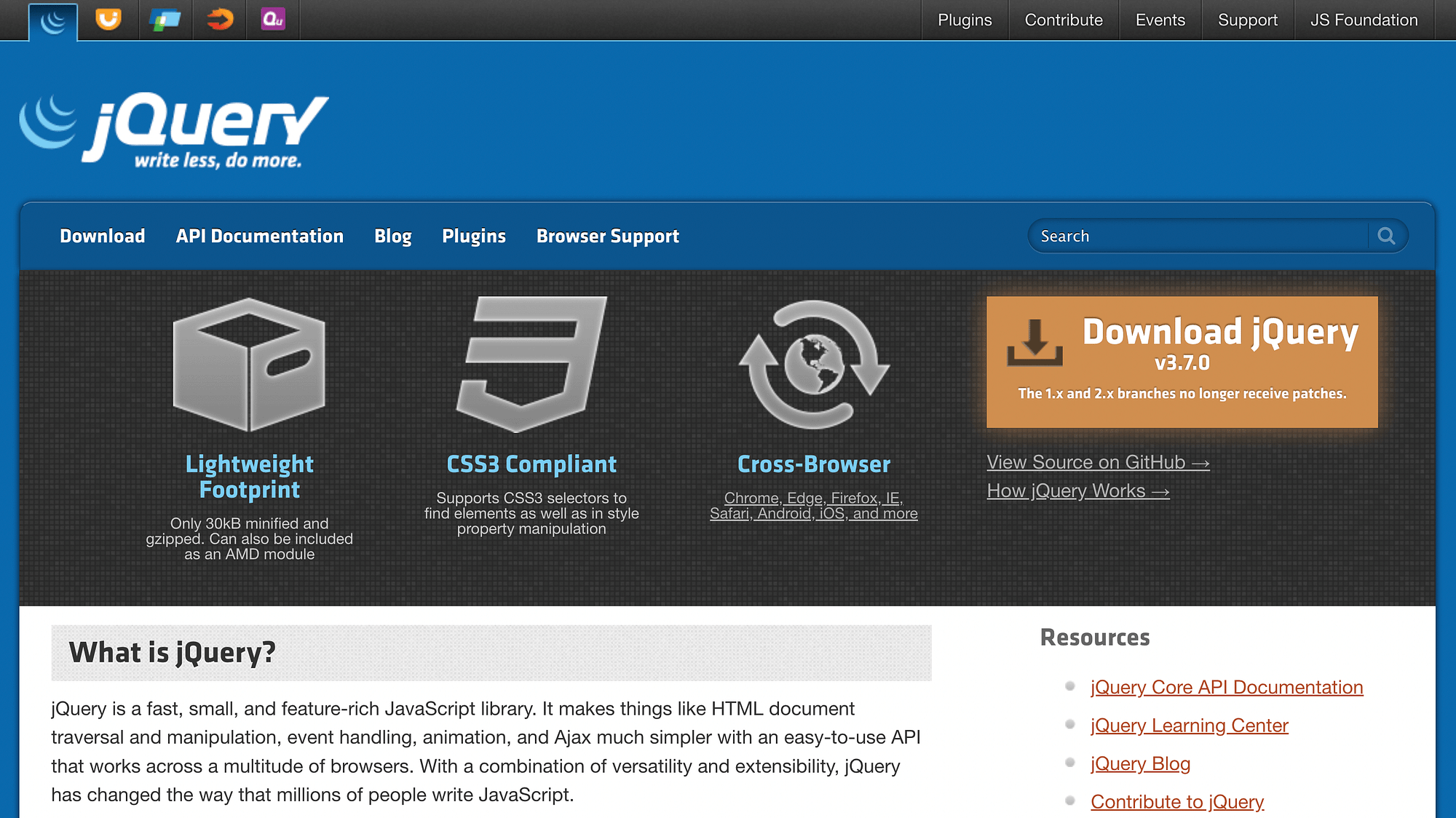The web page for the JavaScript library called jQuery features a clean and structured design. At the top of the page, there is a horizontal, one-inch thick blue bar displaying the jQuery logo styled with a lowercase 'j' and uppercase 'Query', followed by the tagline "Write Less, Do More" in smaller white letters. Above this blue bar is a narrower black bar, about one-sixth the thickness of the blue bar, containing several icons on both the left and right sides, though their functions are not identified.

On the left side of the black bar, there are four icons, while on the right side, there are five tabs labeled 'Plugins,' 'Contribute,' 'Event Support,' and 'JS Foundation.' Below this, there is another navigation bar with links such as 'Download,' 'Blog,' and 'Plugins.'

Dominating the center of the page is a prominent black box featuring a large orange button that encourages users to "Download jQuery version 3.7.0," accompanied by a download icon. To the left of this button, three gray icons are labeled 'Lightweight Footprint,' 'CSS3 Compliant,' and 'Cross Browser,' using blue text.

Towards the bottom of the page, there is an informational section titled "What is jQuery?" followed by a resources list of links positioned at the lower right corner of the page. The layout is designed for easy navigation, helping users quickly find the information and resources they need.